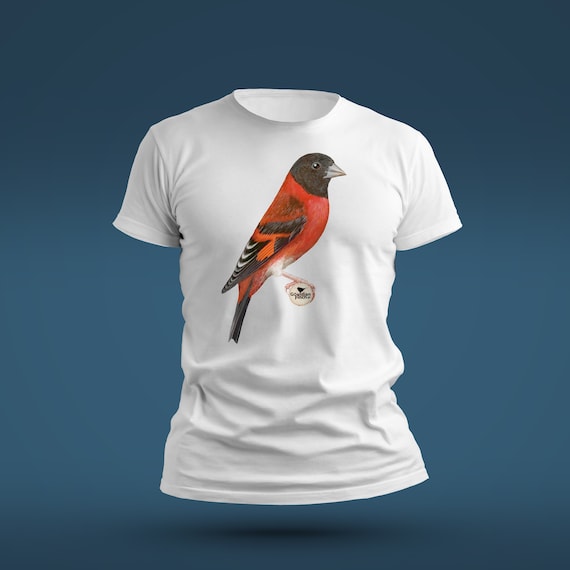This is an image of a white short-sleeve t-shirt with a round neck, displayed against a blue background, appearing as if it's floating. The shirt features a large, photorealistic illustration of a predominantly red bird that spans from the neckline down to the belly button area. The bird, which may be a cardinal, has a brown or black head, black eyes, and a gray or silver beak. The bird’s body is mainly red, including its belly and part of its tail. The wings are adorned with red, black, and white markings, while the tail is black. The bird is depicted standing upright on a tree limb or branch, and beneath its foot, there’s a circle with some words and a small bird illustration, likely representing the logo or brand of the t-shirt. The image focuses on the detailed and vibrant bird illustration, showcasing the contrast against the plain white fabric of the t-shirt.